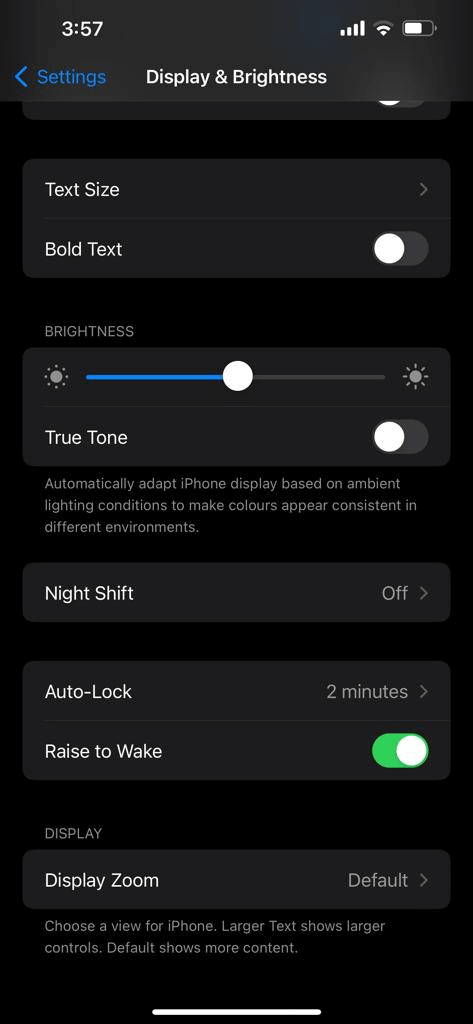**Screenshot of Mobile Phone Settings Page**

The image is a screenshot of a mobile phone settings page with a focus on the "Display and Brightness" options. At the very top, there is a medium gray, blurred header that prominently features a few clear icons and text. On the top-left corner, the number "357" is displayed. Below that, in blue text, it reads "Settings" with a blue arrow pointing to the left, suggesting a navigational element. To the right of this, in white text, the title "Display and Brightness" is visible. 

On the top-right corner, the status icons show five white mobile data bars, a Wi-Fi symbol with two white bars at the bottom and a single gray bar at the top, and a horizontal battery icon indicating roughly 66% charge.

Below this header, the main section of the settings page is displayed over a black background. The section contains various gray, rounded-rectangle buttons, each providing specific setting options. 

1. The top-most section has two rows, each separated by a thin gray line and featuring white text. The first row is labeled "Text Size," followed by an arrow pointing to the right and bold text with a selection button that is turned off. 

2. The next part is dedicated to "Brightness" settings. It includes a slider bar that is blue on the left and gray on the right, with a white circle in the center indicating the current setting. On each end of the bar are white sun icons: one on the left with small dots around it and another on the right with long rays.

3. Below the brightness bar, there is an option labeled "True Tone," with a selection button currently turned off. Beneath this, white text on the black background reads: "Automatically Adapt iPhone Display Based on Ambient Lighting Conditions to Make Colors Appear Consistent in Different Environments."

4. Further down, another gray rectangle contains a single row labeled "Night Shift" with status "off" and an arrow pointing to the right.

5. The next section features two rows: "Auto-Lock," set to two minutes, and "Raise to Wake," with a green toggle switch that is turned on.

6. Following this, white text on the black background states "Display." 

7. The last labeled gray rectangle reads "Display Zoom," currently set to "Default," with an arrow pointing to the right. Below this, white text on the black background explains: "Choose a View for iPhone. Larger text shows larger controls. Default shows more content."